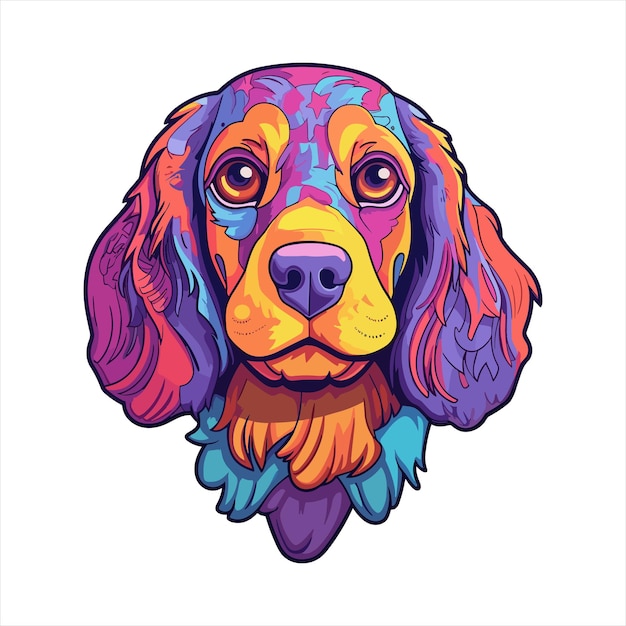This image features a vibrant, highly detailed drawing of a dog's face, resembling a shaggy beagle or hound. The dog is depicted with an array of non-traditional, striking colors. Its nose is a bold purple, surrounded by a blend of yellow and orange hues. The eyes are a mix of golden yellow and orange, with highlights adding a lifelike sparkle. Covering the dog's face are patches of blue and purple, merging into an artistic palette. A distinct purple star is positioned on the upper forehead, adding a whimsical touch.

The ears, one each side of the head, are long, droopy, and fluffy, colored with a combination of purple, red, and burnt orange. The neck fur continues the theme of vibrancy, transitioning from purple to blue and orange in varied sections. The overall design suggests an imaginative and playful approach, perhaps reminiscent of a click-and-paint style, where the artist selected colors at will, creating a lively and eye-catching portrait of the dog's head and part of its neck. The dog faces forward, engaging with the viewer through its large, expressive eyes and colorful, shaggy features.